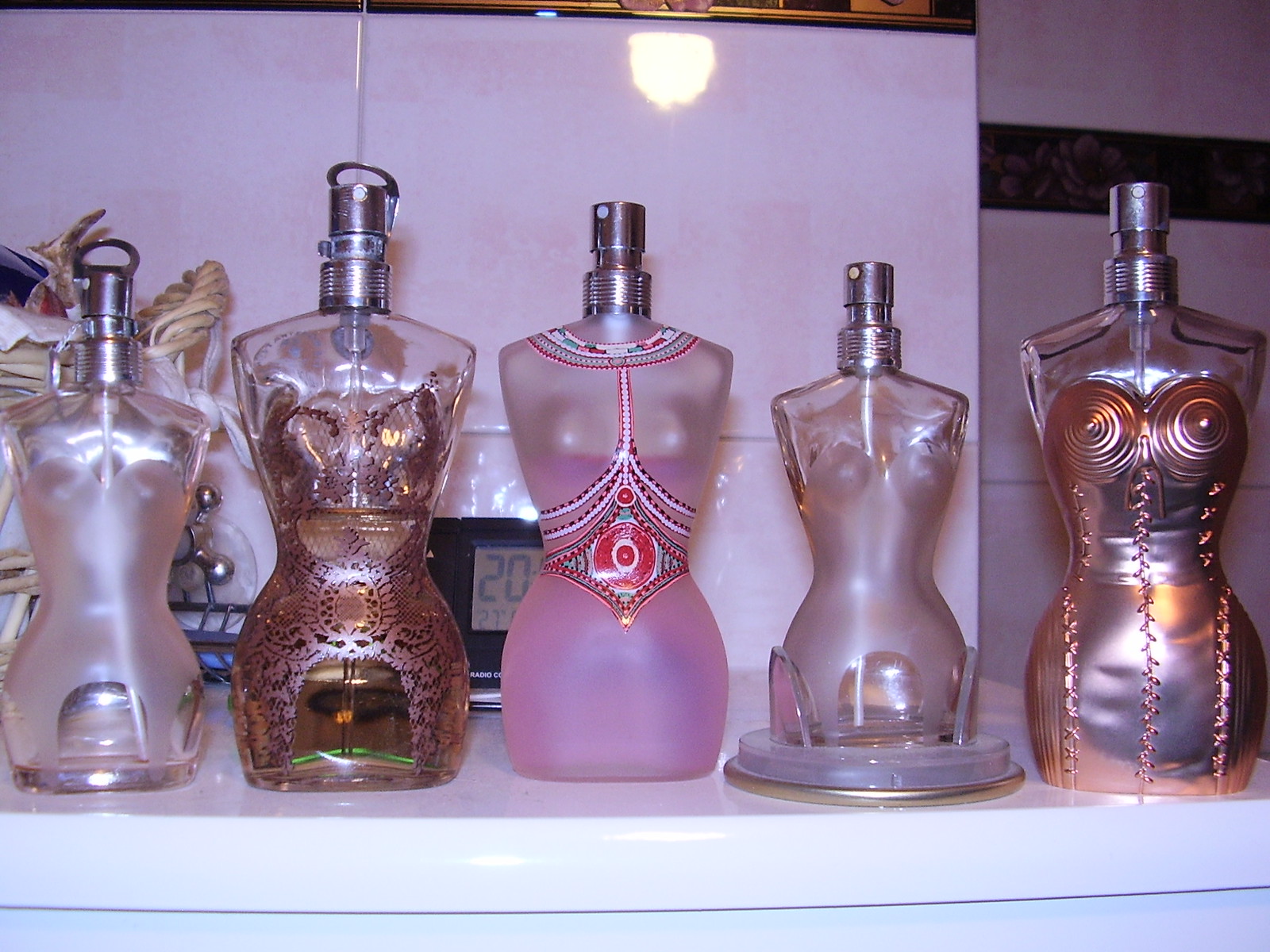The image showcases a display of five intricately designed perfume bottles set on a reflective white countertop. The background features a white screen or wall with a noticeable light reflection, adding to the brightness of the scene. Each perfume bottle is shaped like a woman's torso from the neck to the upper thighs, creating an hourglass silhouette. The bottles are adorned in various types of dressed-up attire, each with unique embellishments and colors:

1. **First Bottle**: Features a misted white dress, mimicking the look of sheer fabric over a clear base.
2. **Second Bottle**: Showcases a lace-inspired dress, slightly larger in size than the first.
3. **Third Bottle**: Wears a pink strapless dress adorned with a multicolored necklace in shades of pink, white, and red. The necklace drapes elegantly under the bust, adding intricate detailing.
4. **Fourth Bottle**: Resembles the first but includes a gold ring detail around a clear stand.
5. **Fifth Bottle**: Displays a rose-gold dress with circular accents on the bust and leaf-like patterns down the torso.

All bottles are accented with silver spritzers, and some dresses include beadwork and metallic hues, reminiscent of high-fashion gowns. The overall aesthetic is luxurious, with the bottles' designs evoking both elegance and a hint of vintage glamour.